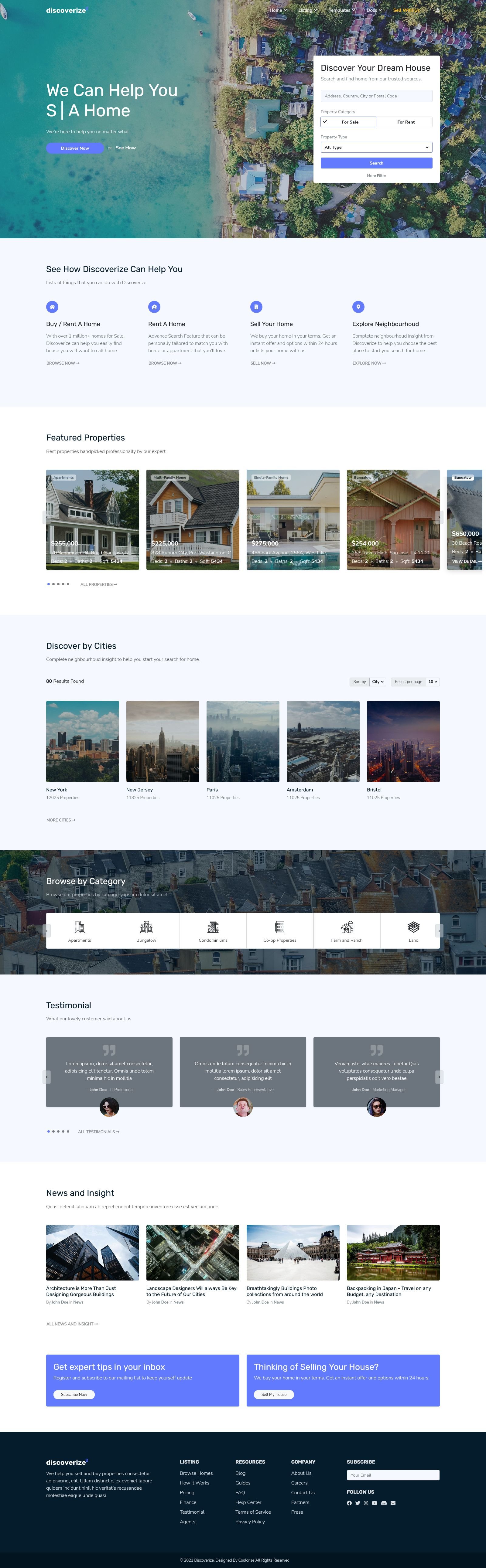At the top left corner of the image, a banner showcases a scene of vibrant aqua-colored water. To the right of this water, a picturesque village emerges, illustrated in an array of blues and purples. On the left side of the water body, there is a white text stating "We can help you," followed by a capital "S," a white line divider, another capital "A," and the word "home." Some smaller, unreadable white text is also present in this section. Below this, a long, rectangular pastel blue button is visible with some white text on it, and to the right, there's more small white text.

Moving to the right, an overlay appears, white and square in shape, seemingly designed to assist users in searching for homes in the area. Beneath this section, a light gray background hosts four distinct paragraphs. Each paragraph's top left is adorned with a circular blue icon containing a white symbol, though the specifics of these symbols are unclear.

The next section transitions into a 'Featured Properties' area with a white background and bold black text. This section displays several properties: on the left, a property with numerous white pillars, a dark blue roof, and a chimney. Adjacent to it is a red house with white trim. Following that, there's a long beige house featuring a pool. Next is a light brown house, and another house that starts but is cut off, leaving it incomplete.

Further down, another light gray background section highlights more properties. The heading here reads 'Discover by Cities,' showcasing various cities with their names in bold beneath each, although the text isn't legible.

At the bottom, another banner is present, displaying several options with gray icons on top. In the top left corner of this banner, 'Browse by Category' is prominently displayed in bold white lettering.